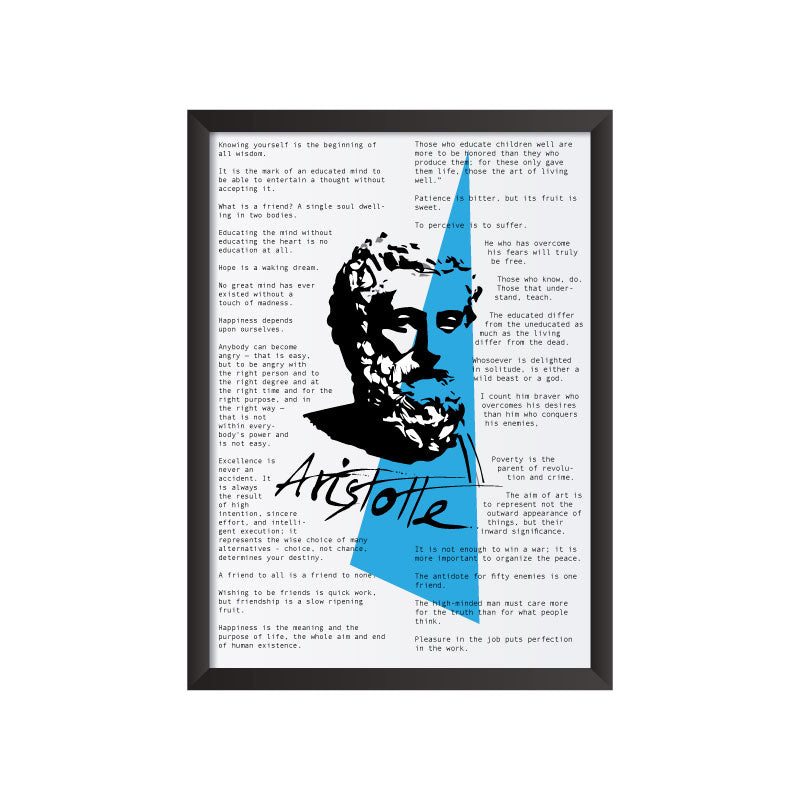This framed print features a white sheet of paper adorned with black typewriter-style text, encased in a black frame. At the center of the piece is a black-and-white image of Aristotle's stone bust, with the name "Aristotle" handwritten beneath it. Quotes attributed to Aristotle are scattered across the poster, including phrases such as "Knowing yourself is the beginning of all wisdom," "To perceive is to suffer," "He who has overcome his fears will truly be free," and "A friend to all is a friend to none." The text is arranged in two columns, structured to resemble the flow of a play or short story. Adding a modern twist to the classical theme, a blue isosceles triangle is superimposed vertically from bottom to top, slightly to the right, partially overlaying Aristotle’s head, giving the poster a unique and artistic appearance.